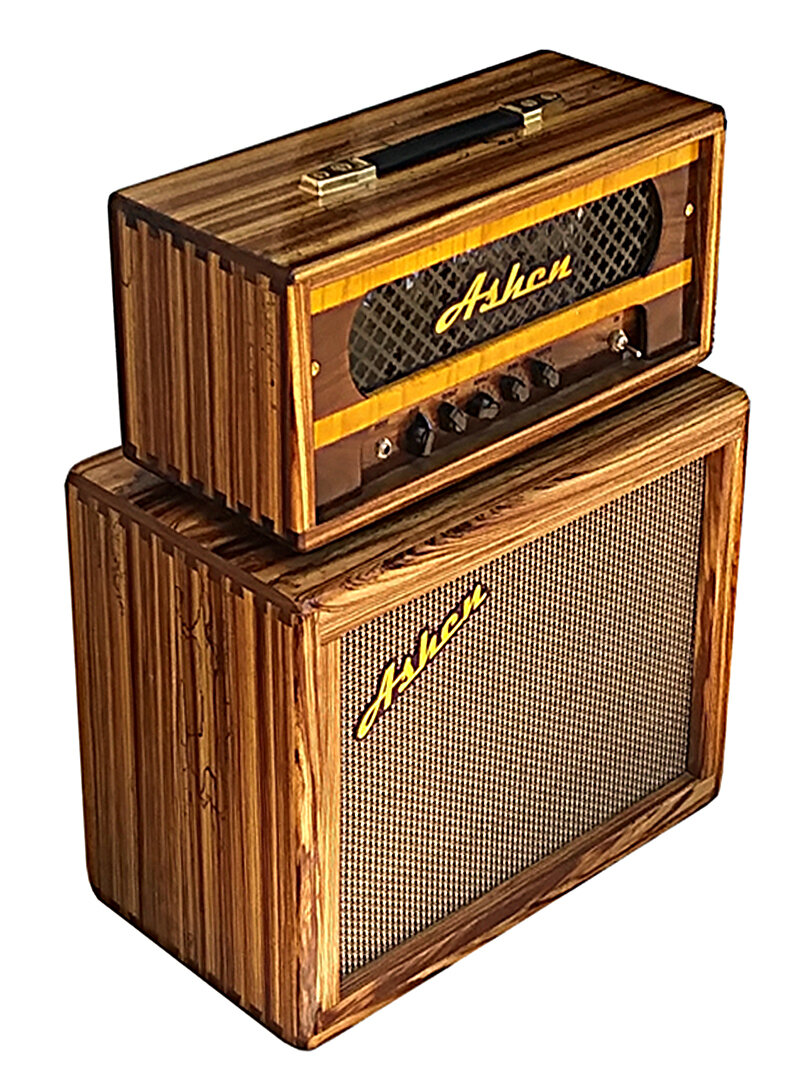The image depicts a vintage audio setup featuring a speaker and a radio, both encased in wood grain cabinets with dovetail joints at the corners, exhibiting a design reminiscent of the 1970s. The larger, lower box is a speaker with a black mesh front grating for sound output, branded with "Ashen" in a diagonal yellow emblem at the top left corner. Stacked above it is a smaller, rectangular radio with a similar wood grain finish. This radio, also branded "Ashen" in the center just above the control area, features five black knobs for adjusting settings like volume and a small silver flip switch for additional control. The radio has a handle on top, distinguished by a black grip with gold accents on each end. The entire setup exudes a classic aesthetic, combining practical audio functionalities with a distinct retro style.